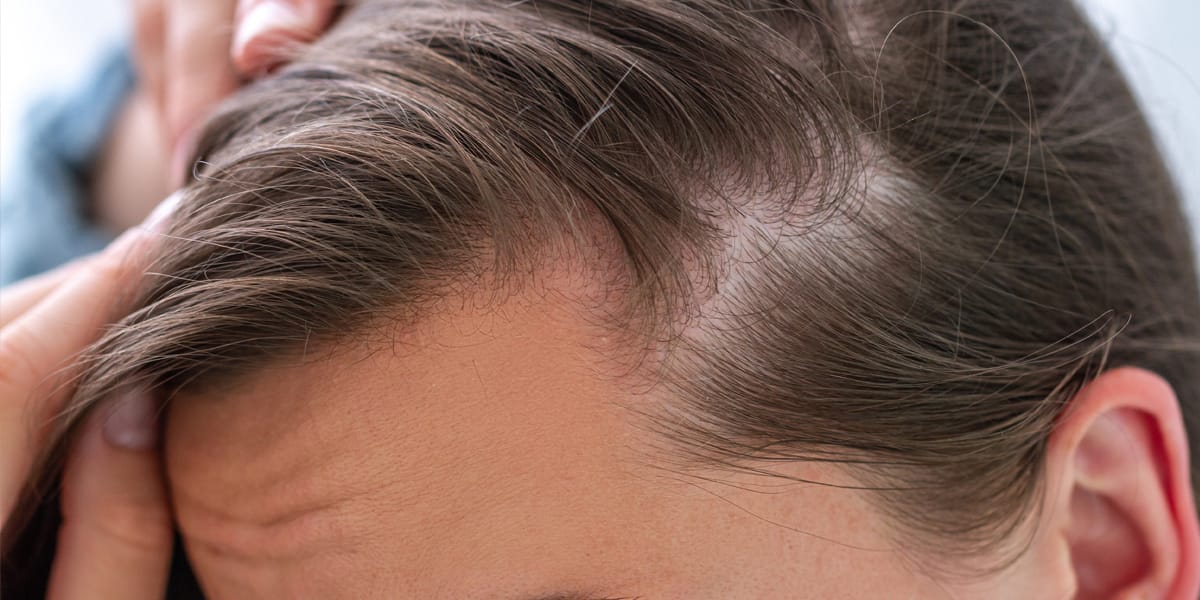The photograph is a close-up shot focusing on the top part of a person's head, specifically from the forehead up to part of the scalp. The image reveals a person with light, tanned skin and dark brown hair being pulled back by their hand, which exposes a noticeably sparse, white area of the scalp. The person's right ear is visible, and part of the left ear is discernible in the far corner of the frame. The hand, blurred slightly, holds the hair over to the left side, while prominent wrinkles run horizontally across the forehead. The photograph is zoomed in and captures detailed textures of the skin and hair, providing no definitive clues about the person's gender. There is no text or background detail, except for a faintly visible light blue sleeve, adding a touch of color to the otherwise focused and intimate portrayal of the person's upper head and scalp.